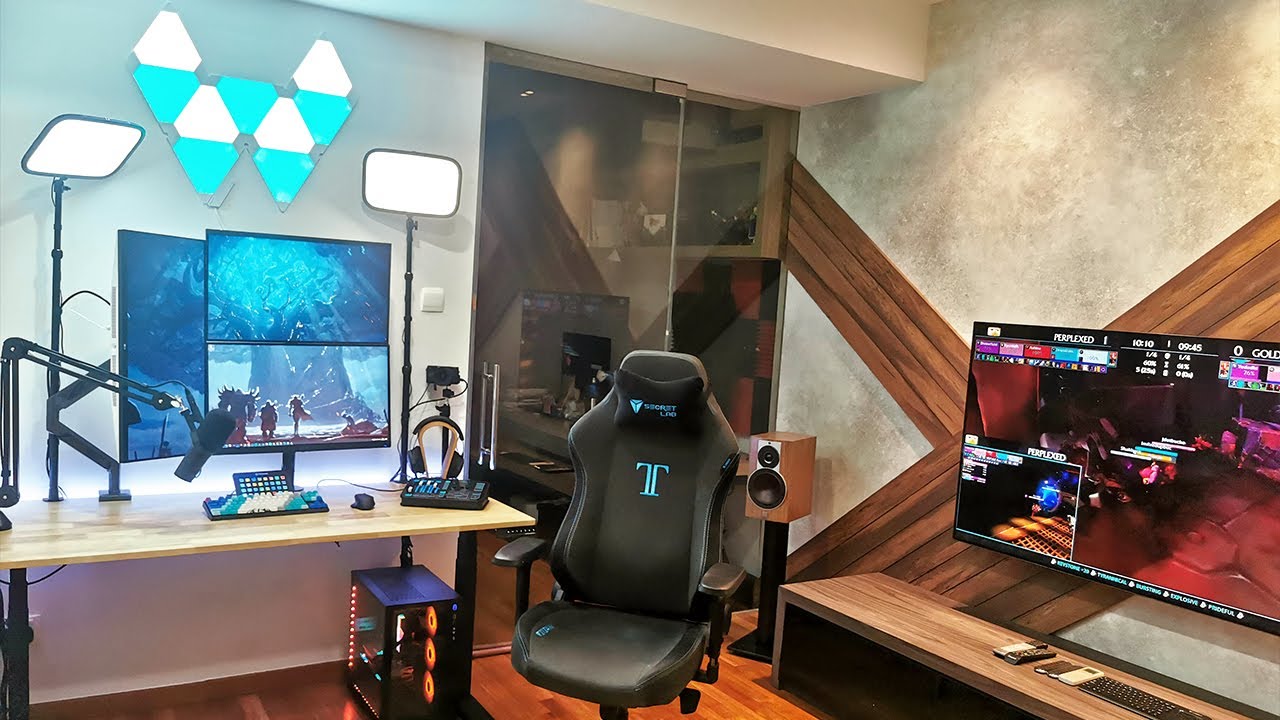This photograph captures an indoor modern gaming room, often referred to as a “gamer's cave.” The main focal point is a high-back black leather gaming chair, featuring a turquoise blue letter "T" on its adjustable headrest, hinting at the brand or model. It is a swivel chair designed for comfort during long gaming sessions. 

In front of the chair is a long rectangular desk with a mix of light brown wood and black metal legs, providing a sturdy yet stylish workstation. Three computer monitors are positioned on this desk in a staggered arrangement—one directly above the other two, creating a multi-functional display setup. The monitors collectively display a gaming scene with characters in front of a grand tree. Below these monitors, there appears to be a modem or router and various gaming accessories, including a microphone and over-the-ear headphones.

Flanking the monitors are two tall black lamps, each with white fluorescent lights that illuminate the workspace evenly. 

On the right-hand side, another long table hosts additional electronic devices including a flat-screen TV which is engaged in a video game, cell phones, remotes, and computer peripherals. A medium brown wooden table beneath supports a keyboard, likely used for managing multimedia outputs.

The room includes diverse wall textures and colors: a light gray wall in one segment, adorned with cross-braced brown wood planks forming an "X" shape, and another section of tan and brown tones. At the junction of these walls, a glass sliding door likely leads to a closet or a different room section. The floor is a reddish-brown wood, adding warmth to the otherwise tech-focused space. Mounted on the floor next to the wall with the TV are freestanding speakers to enhance gaming audio. Overall, the room is skillfully lit and organized to serve as the ultimate gaming setup.